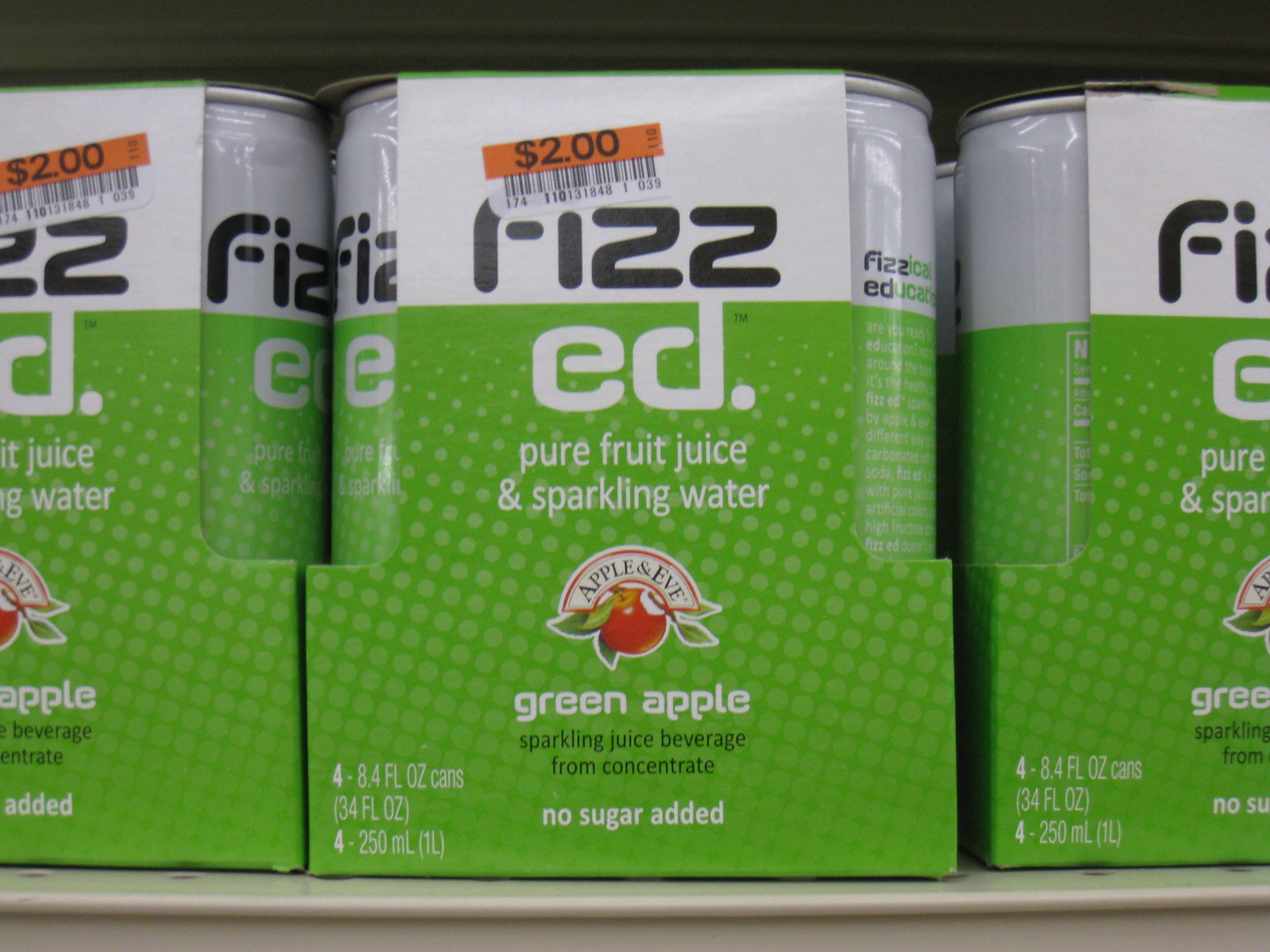A previously packaged set of four 8.4 fl oz cans of Apple & Eve Green Apple Sparkling Juice is depicted. Each can features a red apple with green leaves on the side, with "Green Apple" written in crisp white text at the bottom. The upper part of the cans is white, transitioning to green at the bottom. In the middle, white text announces "Pure Fruit Juice and Sparkling Water." The packaging mentions that the juice was originally concentrated with no added sugar. An orange rectangle prominently displays a $2 price above the barcode. The word "Fizz" is written in black text, followed by "ed" in white text, associating the drink with a fizzy sensation. A symbol is also present at the bottom, enforcing the brand identity.